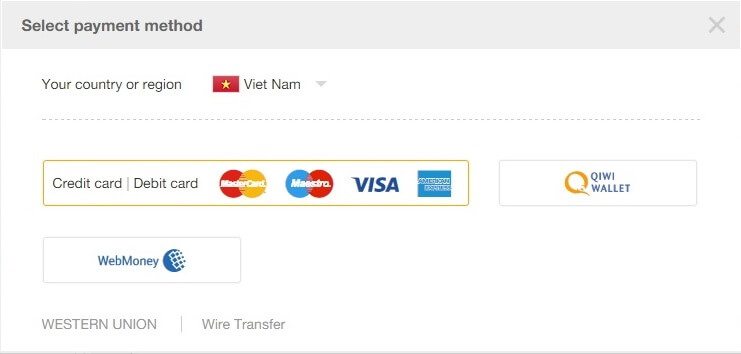The image displays a payment selection screen with a light gray banner at the top. On the left side of this banner, in black text, it reads "Select Payment Method," with "Select" capitalized. On the far right of the banner, there is a light gray 'X' to close the window.

Below the banner, the background changes to white. In the upper left corner of this section, it says "Your Country or Region" with "Your" capitalized. The selected country is Vietnam, indicated by the red flag with a yellow star and the text "Vietnam" beside it, written as "V-I-E-T, Nam" with "V" and "N" capitalized. A light gray arrow pointing downward suggests more options are available.

A dotted gray dividing line separates different payment options. The first bar on the left lists "Credit Card" followed by a gray horizontal line, and "Debit Card," with "Credit" and "Debit" capitalized. Below this, there are four logos: a MasterCard logo with a red and yellow circle and white text; a Maestro logo with a blue and red circle and white text; a Visa logo with capital blue letters in a white box; and an American Express logo with blue letters in a blue box.

To the right, another box displays "QIWI Wallet" with a large capital "Q" in gold next to the text. Below the Credit and Debit Card box, there is "WebMoney" with "W" and "M" capitalized, followed by a round logo with a white mesh-like design.

At the bottom, there are options for "Western Union," written in all capital letters in gray with a horizontal dividing line, and "Wire Transfer," also in gray with capital "W" and "T."